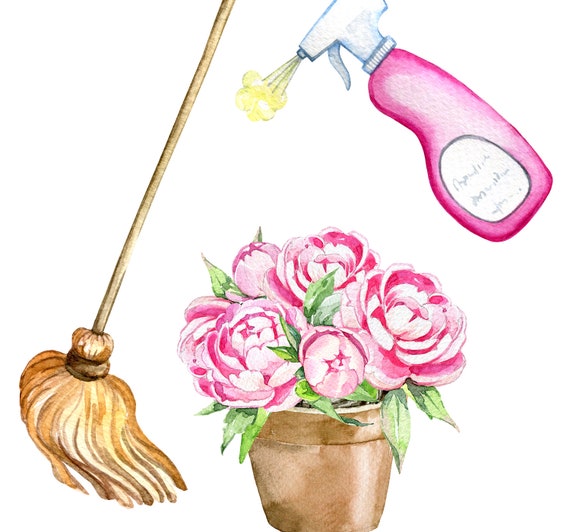This image is a charming watercolor illustration set against a white background. At the center bottom, there is a brownish-tan flower pot filled with pink and white begonias, accompanied by some green leaves. To the left, an old-fashioned mop with a wooden handle and a cloth mop head, reminiscent of the one from "The Sorcerer's Apprentice," stands upright. In the top right corner, a pink spray bottle with a white label and a white spray top angles downward. The bottle emits a yellow puff, suggesting moisture being sprayed. Overall, the illustration combines household items with floral beauty in a delicate watercolor style.